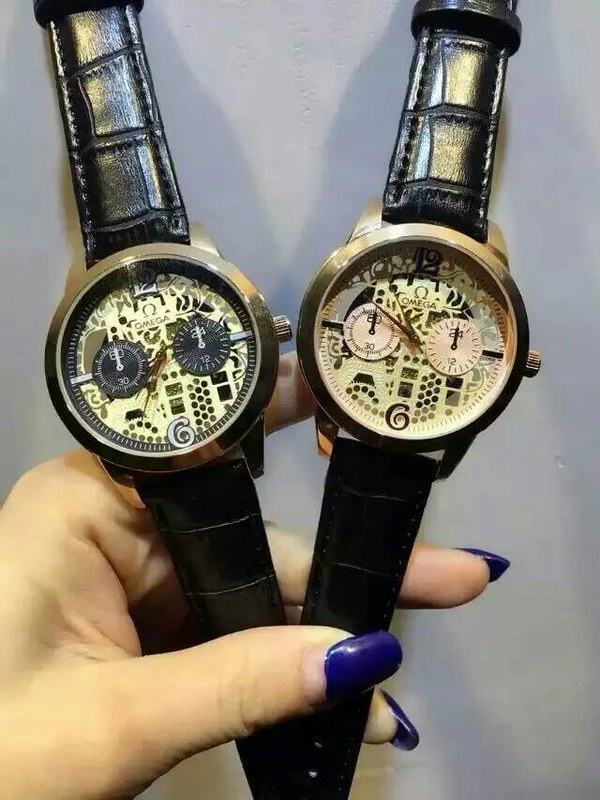This photograph depicts a woman's left hand, with light-colored skin, emerging from the bottom left corner of the image, creating a somewhat surreal effect as her fingers appear unusually long and misshaped. Her nails, painted in a deep navy blue color, are notably elongated and slightly rounded at the tips, revealing growth from the cuticles. She is holding two wristwatches, each featuring well-worn black leather straps with visible signs of wear. Both watches are branded "Omega" and display large dials with intricate designs. The watch on the left has a bluish-green background with two inner circles bearing white numerals "60" at the top and "30" at the bottom, and an hour and minute hand. The watch on the right has a light green and pink background with two beige circles marked "24" and "12." Both timepieces have decorative, gold-trimmed faces and small knobs on their sides. The distorted nature of the image enhances the unusual, stretched appearance of the woman's hand and fingers, lending an intriguing and somewhat bizarre quality to the photograph.